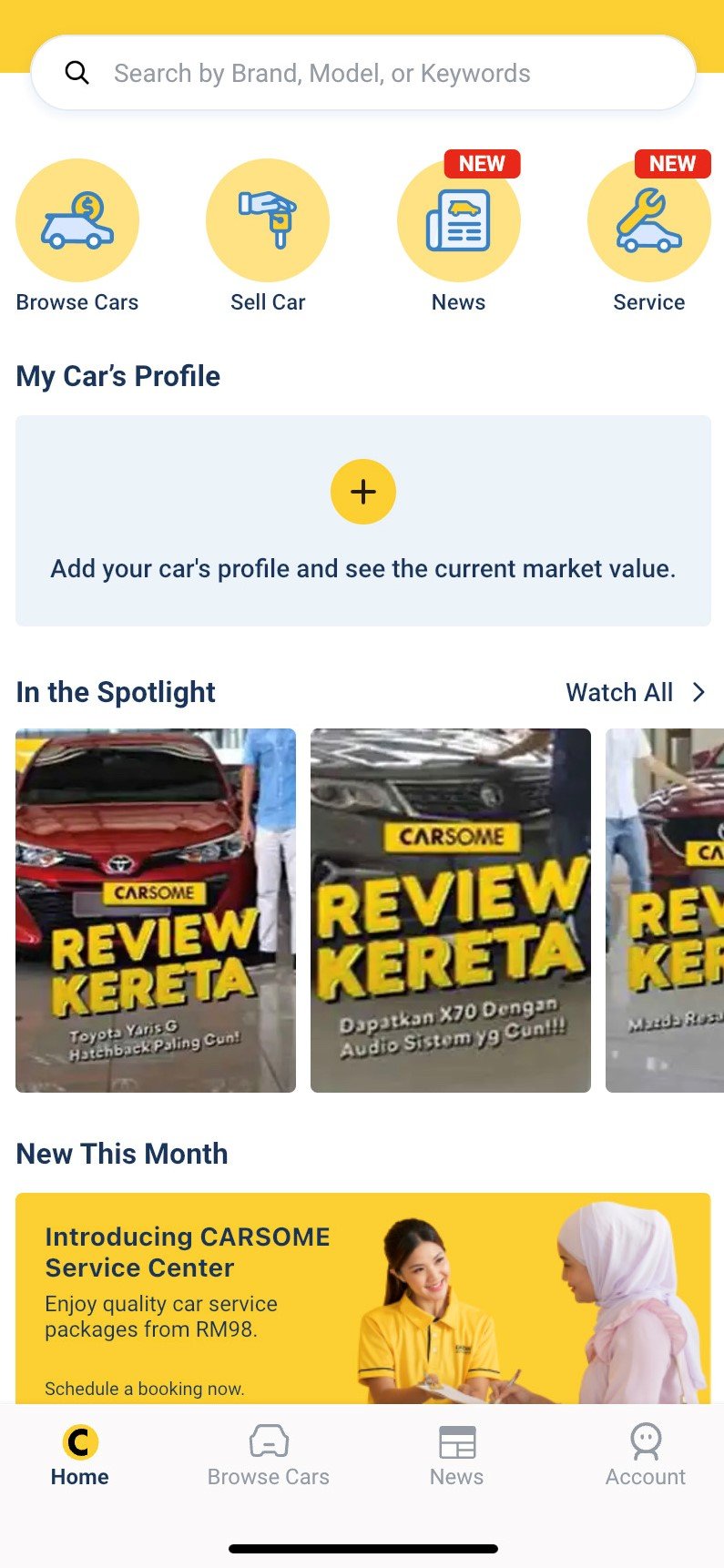A detailed screenshot of a car purchase website's mobile interface, predominantly in English, yet it features design elements suggesting a Southeast Asian market, possibly the Philippines or Malaysia. At the bottom of the screen, a customer and an attendant engage in what appears to be a service interaction. At the top, a search bar is prominently displayed, followed by menu options including "Browse Cars," "Sell Car," "News," and "Service." Additionally, there is a section labeled "My Car's Profile" with a plus sign, indicating the option to add a car's profile and view its current market value. 

Below this, a section titled "In the Spotlight" features clickable content such as reviews for the Toyota Yaris G Hatchback and other vehicles. Another area called "New This Month" introduces the Carsome Service Center, highlighting Troy Quality Car. The screen's layout is completed with a navigation bar at the bottom containing shortcuts to "Home," "Browse Cars," "News," and "Account."

The site’s branding is indicated by the name "Carsome," suggesting it plays a significant role in the content and services offered.